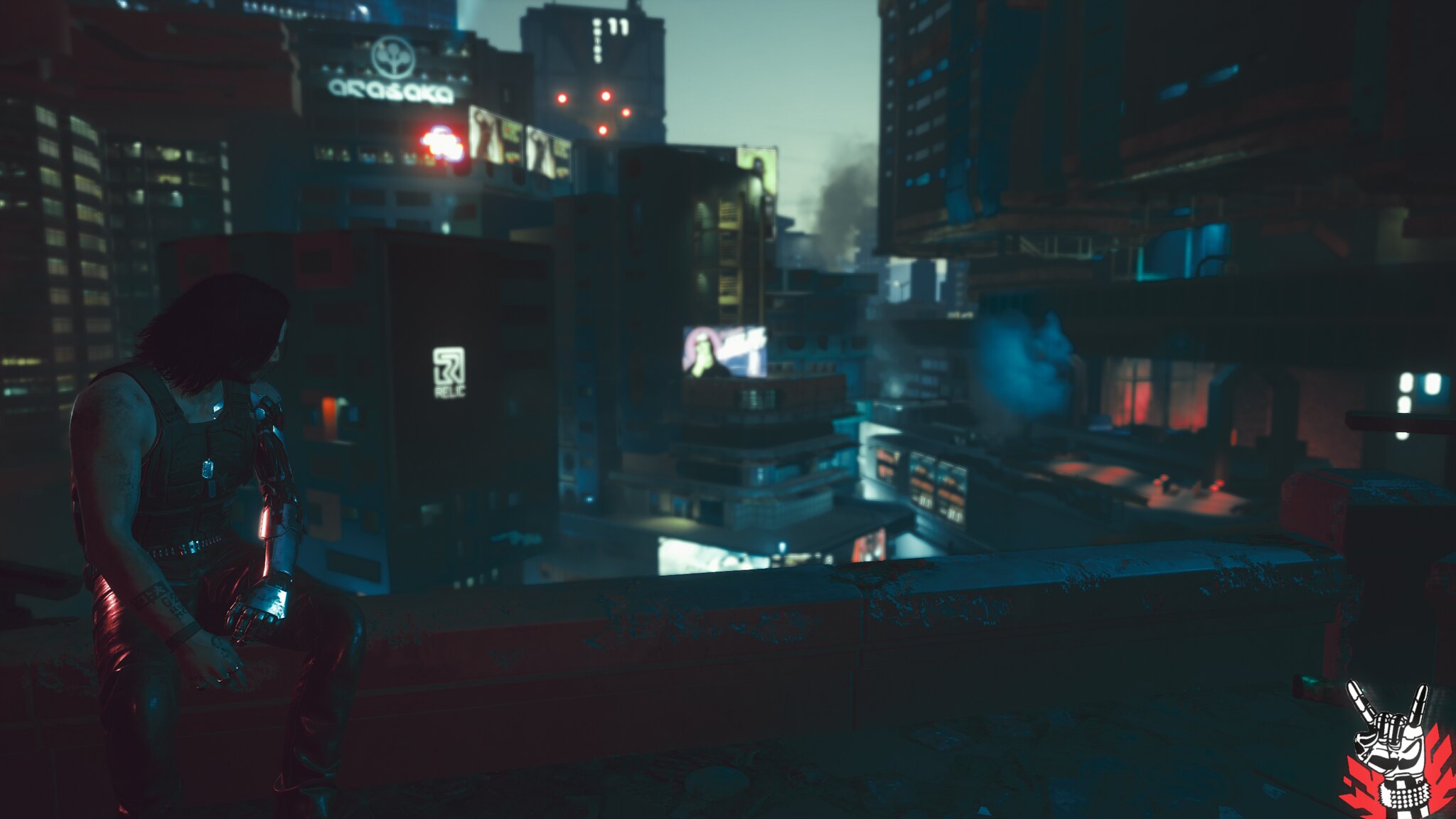In this captivating image from a post-apocalyptic movie scene, a muscular man with shoulder-length black hair sits on the edge of a tall building, gazing out over a devastated cityscape. His attire includes a black muscle shirt and leather pants, and he sports a detailed tattoo on his right arm. Notably, his left arm is a mechanical prosthetic, adding to the futuristic, dystopian atmosphere. The city below him is illuminated by various lit signs, although the names on the buildings are indiscernible. Smoke billows from several structures, indicating recent destruction, and the overall setting evokes a resemblance to a ravaged New York City. In the bottom right corner of the frame, another muscular arm emerges, with fingers forming a peace sign, suggesting a message of resilience amidst the chaos.